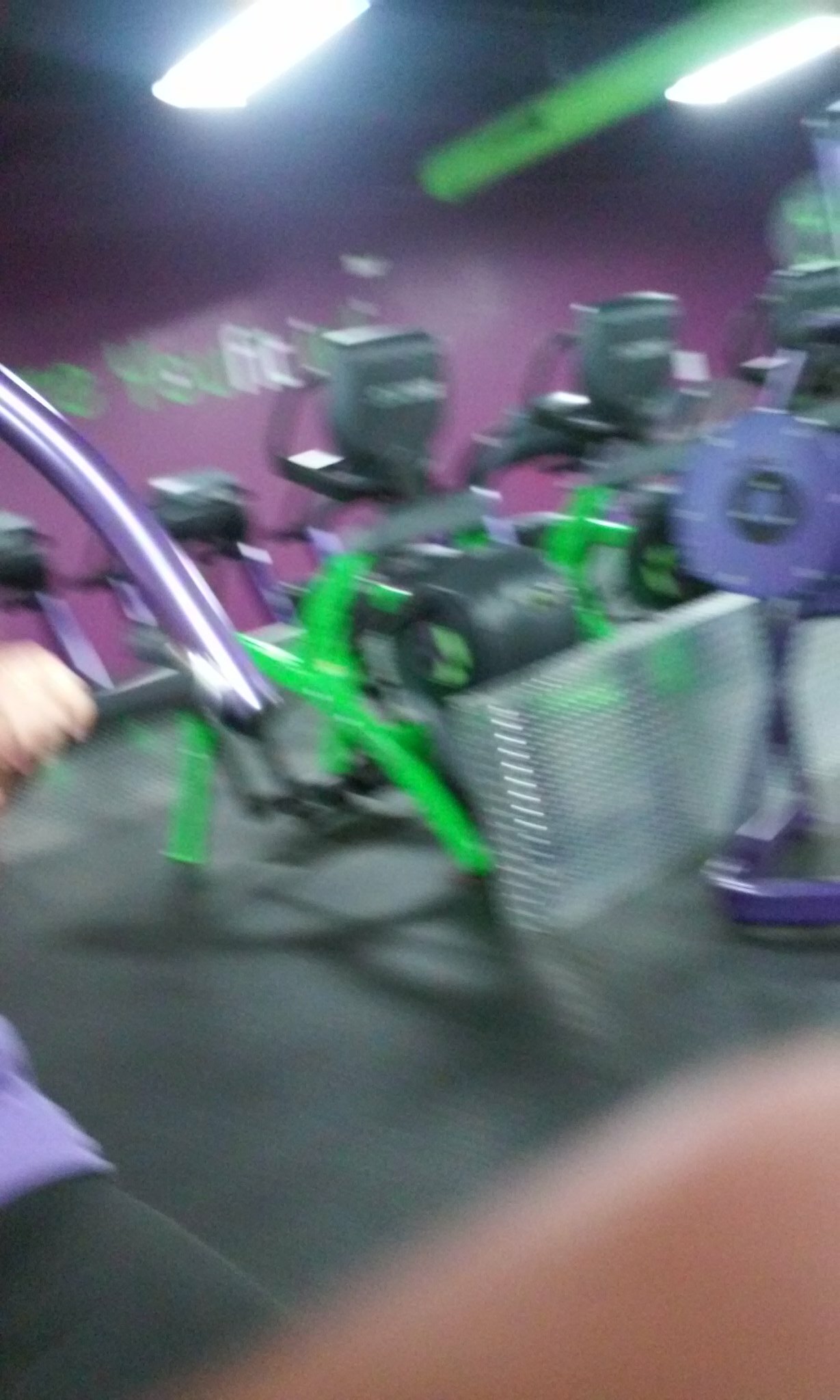A blurry photograph captures the indoor area of a public gym. The back wall is painted in a deep purple hue, adorned with green and white lettering that is difficult to decipher due to the image quality. Long, white ceiling lights illuminate the space, and a green pole-like structure hangs prominently from the ceiling. In the bottom right corner, a finger partially obstructs the view. The main focus is on several types of exercise machines, possibly bicycles or treadmills, arranged in rows. None of the five visible machines are occupied, highlighting the emptiness of the gym at this moment.